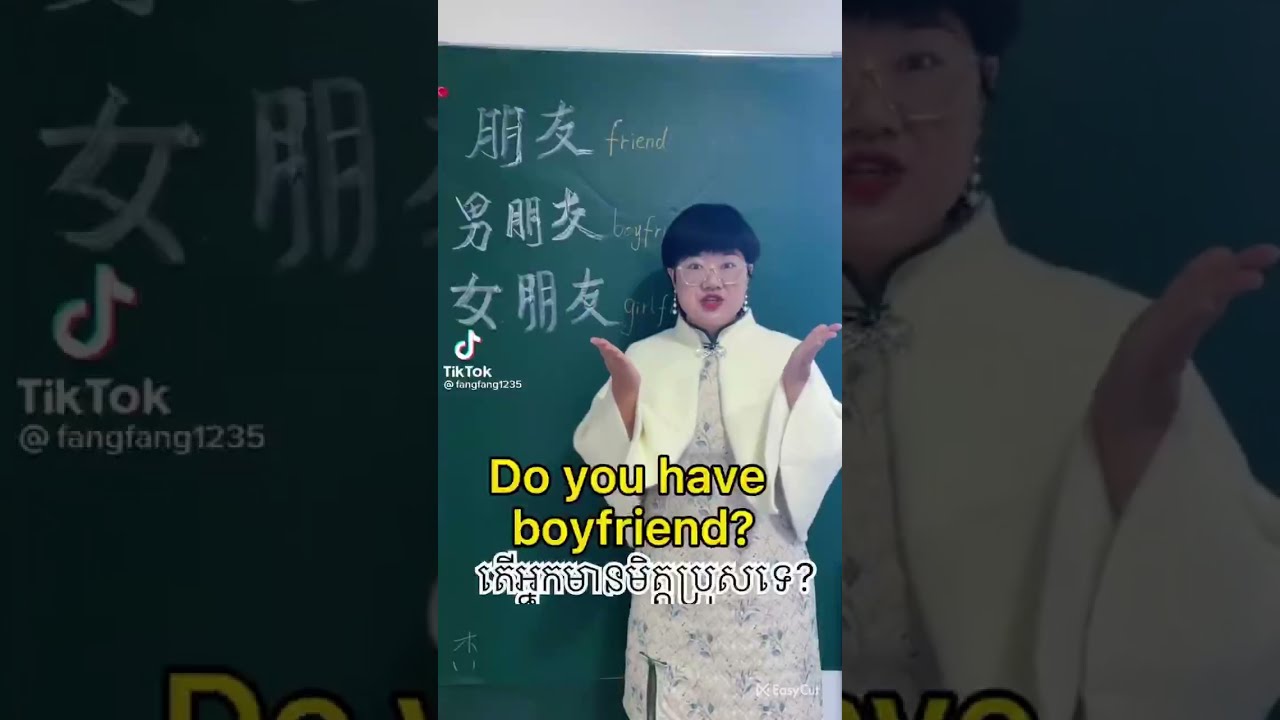This image is a horizontally arranged, three-panel photograph featuring a female teacher who appears to be of Asian descent. The primary focus is the central panel, which showcases a close-up of the teacher standing in front of a green chalkboard with her hands slightly raised in a gesture that suggests surprise or emphasis. The woman has short, dark brown-black hair styled in a bowl cut, wears eyeglasses, and is adorned in a white cardigan over a gray dress with floral patterns. She accessorizes with dangly earrings and red lipstick.

The chalkboard behind her displays three rows of white symbols and corresponding English words: "friend," "boyfriend," and "girlfriend." There are additional indecipherable symbols beneath these terms. The words "you have boyfriend?" are prominently displayed in bold yellow letters with a black border across the center of the image.

On the left side of the image, a faded, close-up version of one of the symbols on the chalkboard appears, along with the TikTok logo and the username "fang_fang1235". The right side of the image features another close-up, slightly faded image of the woman, emphasizing the details of her face and attire.

This composite image appears to be a screen capture from a TikTok video, possibly focused on language teaching or a cultural lesson, as suggested by the bilingual text on the chalkboard.